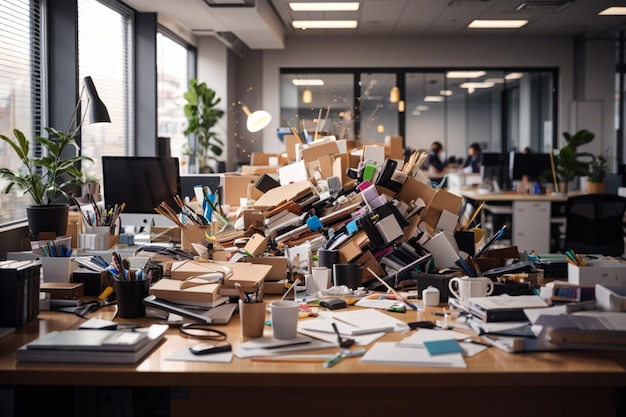This indoor daytime photograph depicts a cluttered office setting. In the foreground, there's a brown wooden desk, which transitions from being somewhat organized on the left and right sides—holding papers, pencils, and other standard office items—to an utter chaos towards the center and back. Piled in a giant heap where the occupant should be sitting are an assortment of cardboard boxes, office folders, packages, black plastic containers, and various office supplies, giving the impression that deliveries and shipments have been left unattended for quite some time. To the left of this clutter rests a lamp and a small green plant in a black pot, and there's an Apple iMac display. Behind the desk, to the left, three large windows with horizontal blinds offer a slight view outside, confirming it's daytime. Recessed ceiling lights are spread throughout, illuminating the room, which features white drop-down ceiling panels. There are indications of more organized office space beyond this chaotic scene; people are working in the background, though their faces are blurred. The larger room also includes potted plants and likely serves as a conference area, with large windows providing visibility into another room. Overall, despite the desk's disarray, most of the office maintains a clean and orderly appearance.